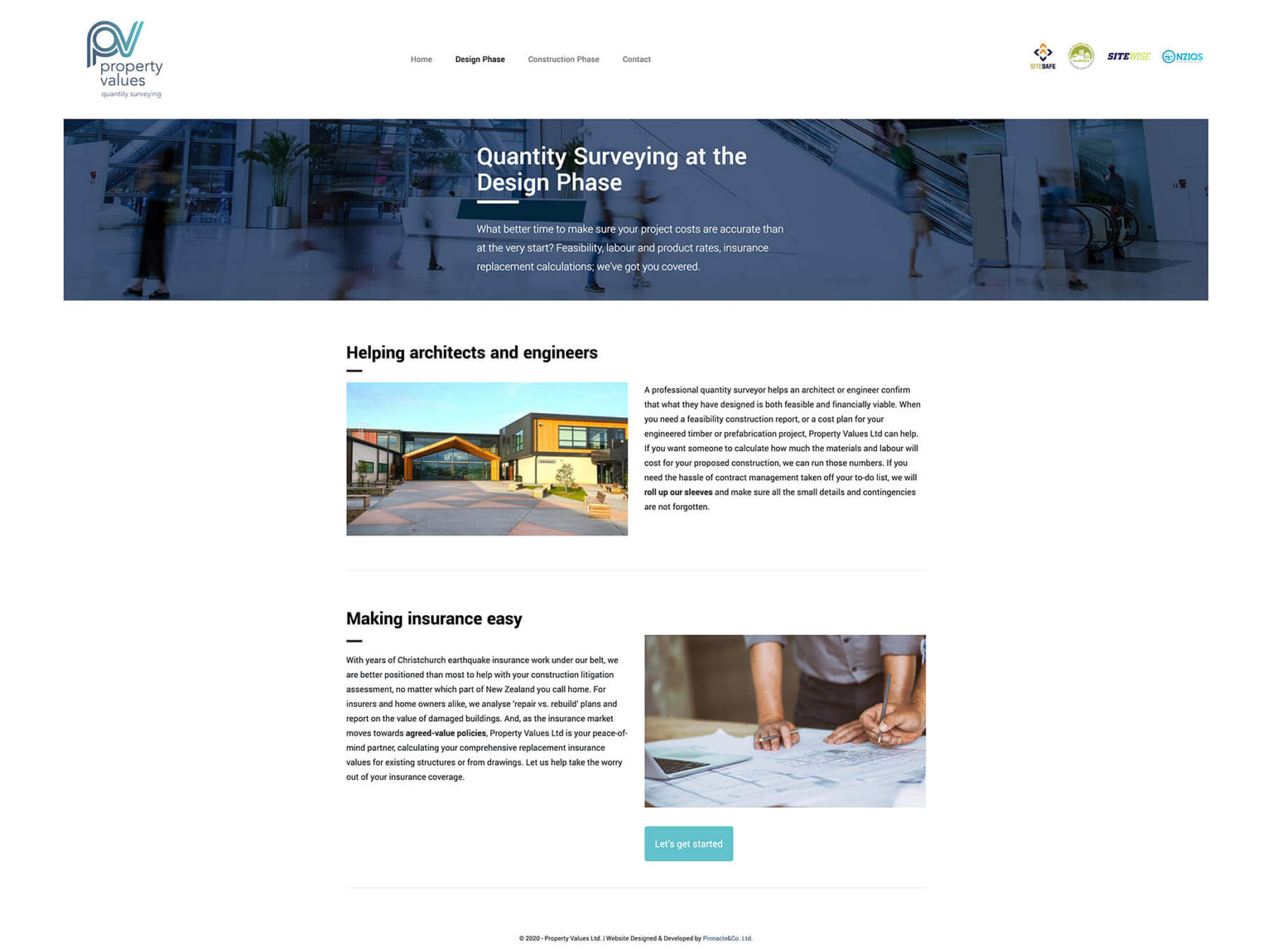This webpage is focused on providing tools and information for accurately assessing property values during the design phase of a project. The introductory section emphasizes the importance of ensuring precise cost calculations at the beginning of a project. It highlights key considerations such as labor and product rates, insurance, and cost readjustments, affirming that the platform covers all these aspects comprehensively.

At the bottom of the introductory content, there is an image of a modern building, accompanied by the phrase "Helping Architects and Engineers." Although there's a paragraph of text next to the image, its font size is too small to read easily.

Further down, the webpage includes a section titled "Making Insurance Easy," which also has an accompanying paragraph with text that's similarly difficult to read. Beside this section, there's a photograph depicting an architect examining detailed plans laid out on a table, conveying a sense of meticulous planning and focus.

Finally, the webpage concludes with a call to action that reads "Let's Get Started," paired with a prominent button designed to initiate user engagement. The overall theme underscores the importance of early cost management, support for architects and engineers, and the facilitation of insurance processes.